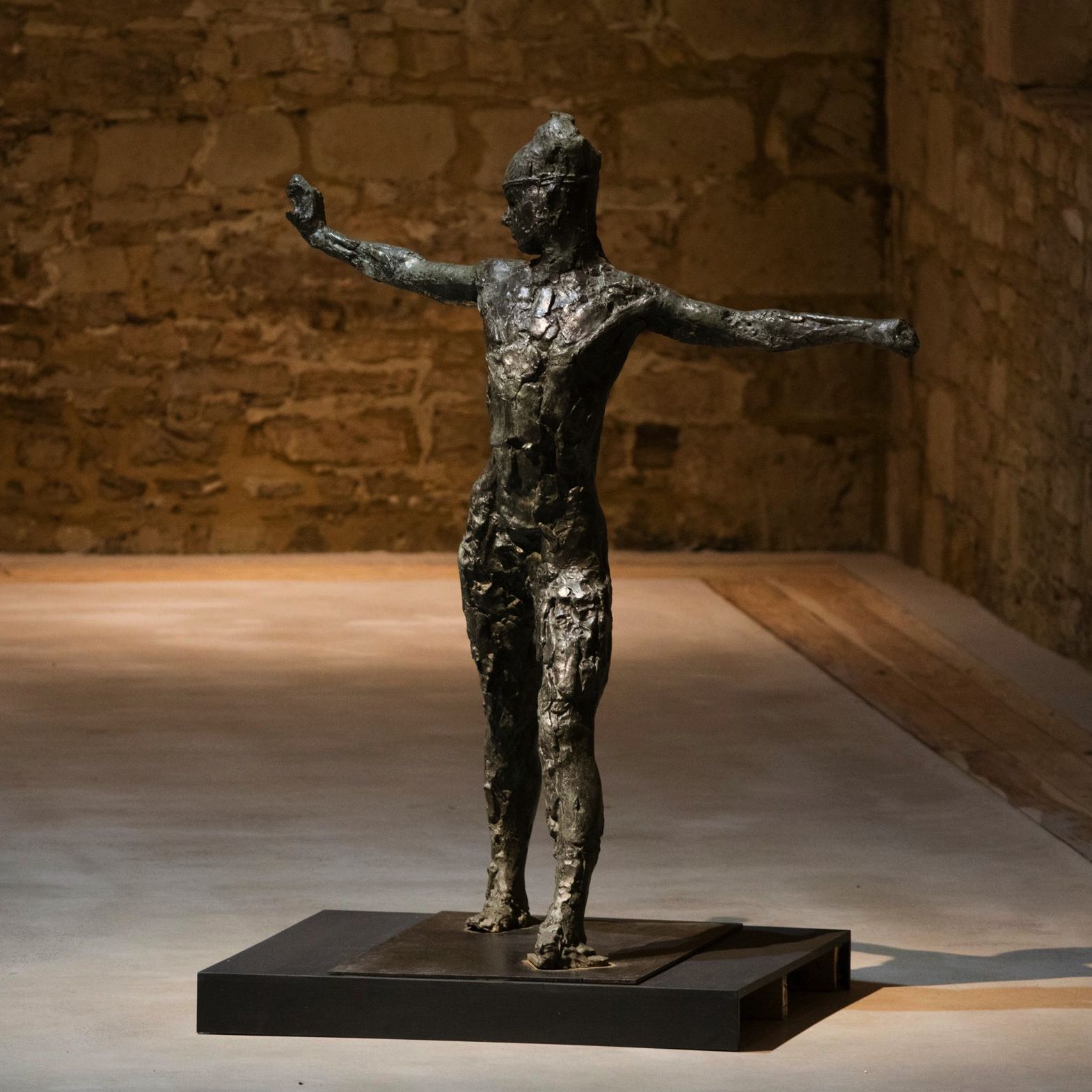This photograph captures a dark bronze sculpture of a human figure standing on a black wooden plinth in the center of a large room. The figure, with its arms outstretched, is depicted with a rough and bumpy texture that reflects light from a source positioned above and to the left. The figure's body faces the camera while its head, adorned with a tight-fitting helmet, turns to the right. The sculpture's legs are positioned one in front of the other, adding a sense of movement to the piece, and the details of the clothing are abstract and indistinct, with the surface marked by creases and folds. The room features a floor comprised of both light brown wood and sections of concrete and brick, leading up to two stone walls at the back that diverge at an angle. The walls are constructed from irregular stones of varying shades of brown and gray, adding to the textured and earthy environment of the space.